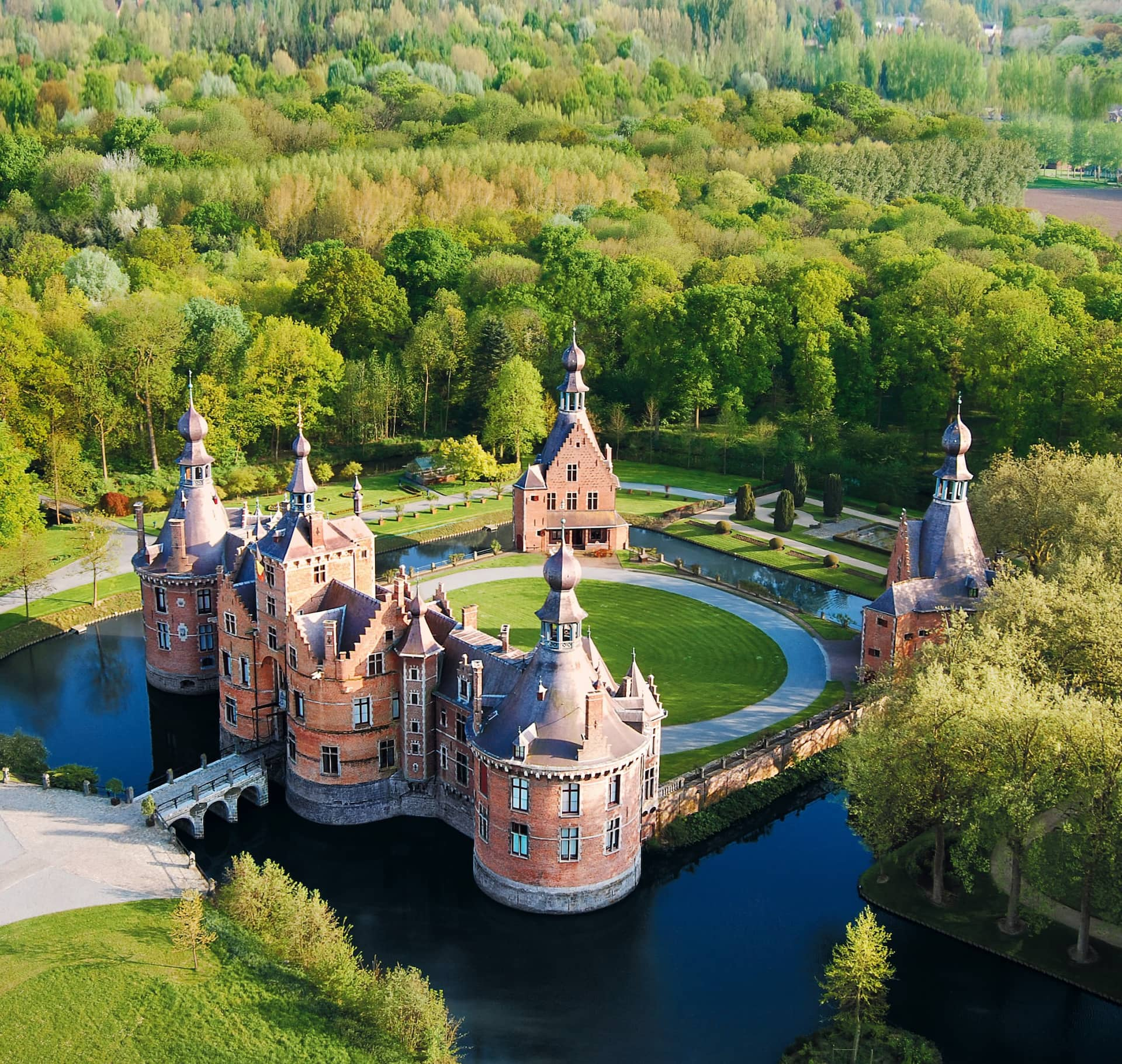This aerial photograph captures a breathtaking, lush landscape dominated by thick green trees and shrubbery. Amidst this verdant expanse lies an exquisite castle, constructed from pinkish-red brick with tall, pointed steeples. The castle complex consists of multiple brick buildings, at least four main sections, each adorned with decorative and pointy roofs. A distinctive small white bridge spans a very dark blue body of water at the front, creating an elegant entrance to the castle grounds.

In the immediate foreground, a neatly kept green lawn is bordered by a white pathway that forms a perfect circle, encircling the grassy area. This intricate pathway and manicured lawn lie between the multi-structured castle and other auxiliary buildings, each featuring its own steeple. 

Beyond the castle and its orderly grounds, the backdrop is a continuous stretch of dense, vibrant greenery made up of rows upon rows of trees that emphasize the serene and secluded nature of this majestic estate.